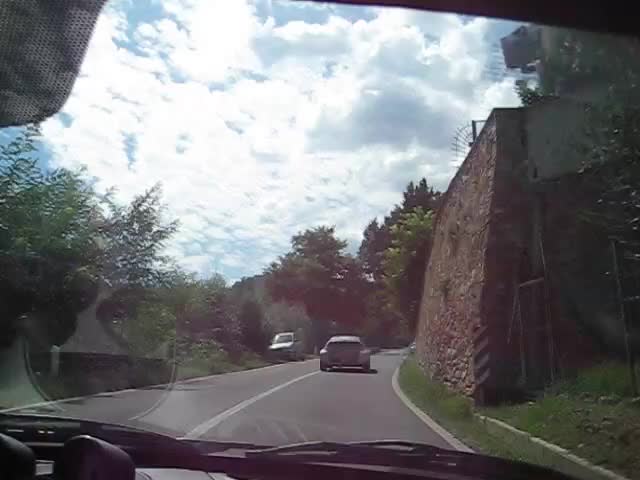This color photograph captures a scenic drive from the passenger side of a vehicle. The image, taken through the windshield, reveals a dashboard with off-position windshield wipers. The sky is a blend of blue with light and gray clouds, setting a serene atmosphere. The road ahead is gray with white dividing lines, flanked by a reddish rock cliff on the right with green grass beneath it. In front of the vehicle, there are trees lining both sides of the road. Two cars are visible: one driving ahead and another, possibly a van or truck, parked on the grassy shoulder of the opposing lane. The dashboard’s reflection faintly appears in the window, enhancing the perspective of being inside the vehicle.